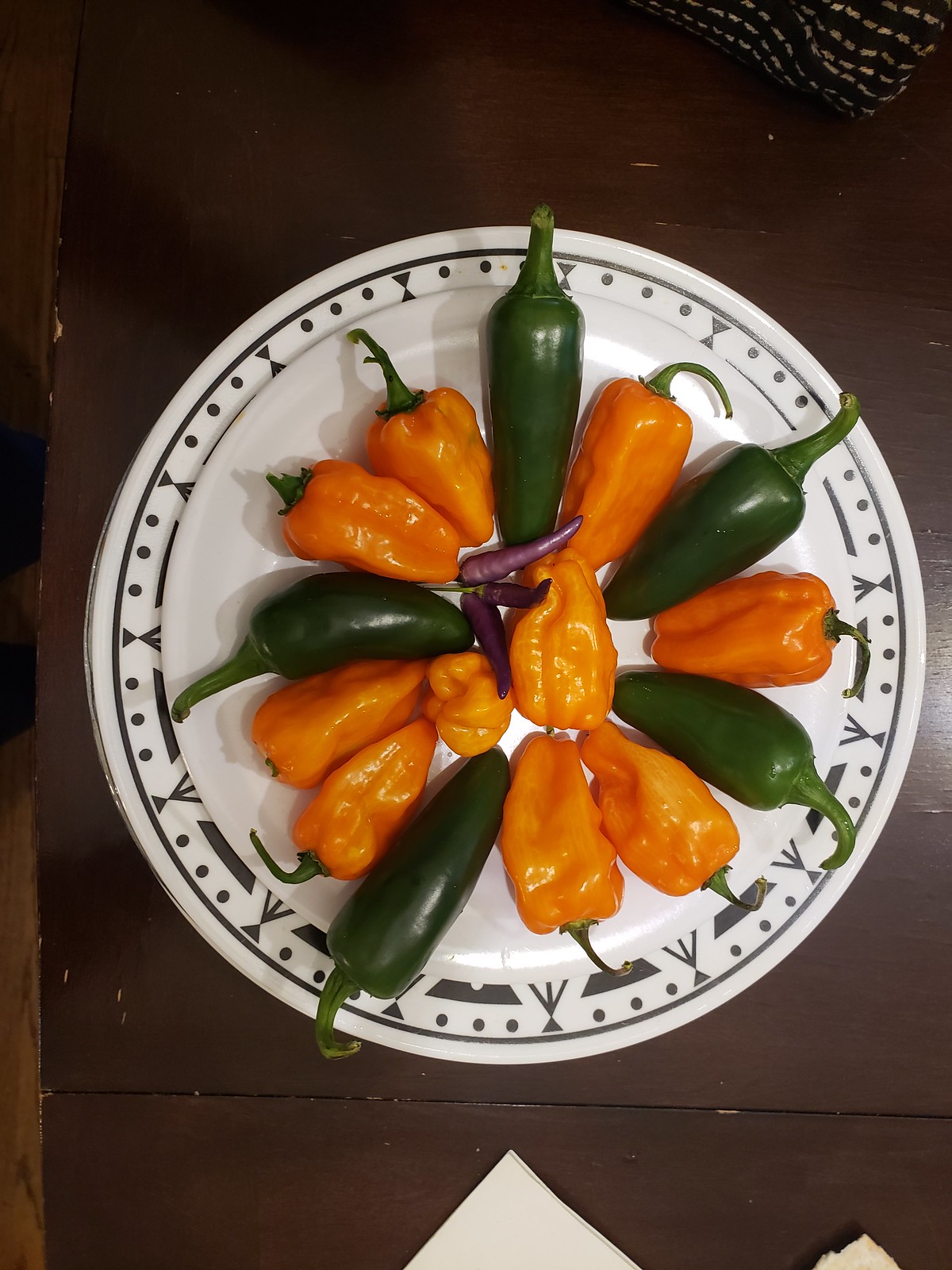This photograph captures a beautifully arranged plate of peppers set on a dark wooden table. The white plate features a black and green dotted design interspersed with triangles and hourglass shapes. Center stage are the vibrant peppers: five smooth green peppers, possibly jalapenos or serranos, around which ten wrinkled orange habanero peppers are meticulously placed, adding a burst of color. Nestled among them are three small, elongated purple peppers, possibly beets. The intricate design of the plate and the vivid array of peppers—dark green, orange, and purple—create a visually striking composition, emphasizing the fresh and varied produce. In the bottom corner, a white napkin slightly peeks into the frame, adding a subtle element to the setup.